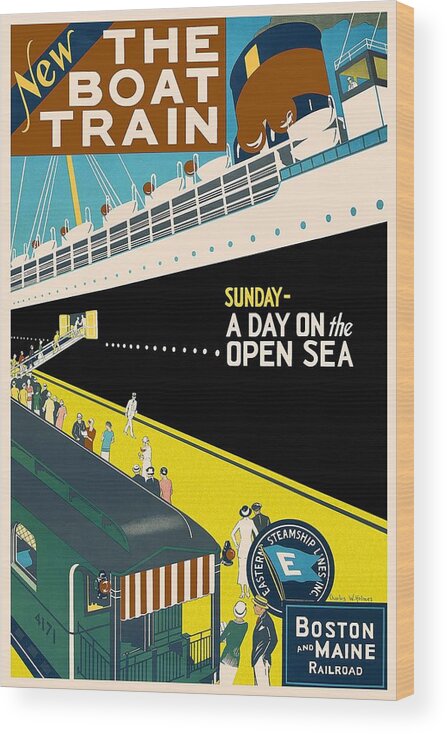This image is a detailed vintage advertisement for train travel, prominently featuring a new service called "The Boat Train." In the upper left corner, a brown rectangle with white letters displays the title, and the word "NEW," written in yellow and slanted upward, conveys excitement. The background has a graphic illustration of a large cruise ship with a black hull and a white top. Billowing from the ship's smokestack is reddish-brown steam. Text on the black section of the ship reads "Sunday" in yellow and "A Day on the Open Sea" in white. 

To the left, the poster shows passengers on a yellow dock ramp leading to the ship, transitioning between the train and the vessel. The ground area where people are walking is also yellow. A green train, distinct with its dark green and black body and numbered 4171, stands at the lower part of the image. A woman in a green top and white hat is depicted hanging off the train. 

At the bottom right, white letters state "Boston and Maine Railroad" next to a circular logo of Eastern Steamship Lines Incorporated, featuring a flag with the letter "E." The poster predominantly uses colors such as black, white, yellow, brown, green, blue, and some pink accents, likely dating back approximately 89 years.